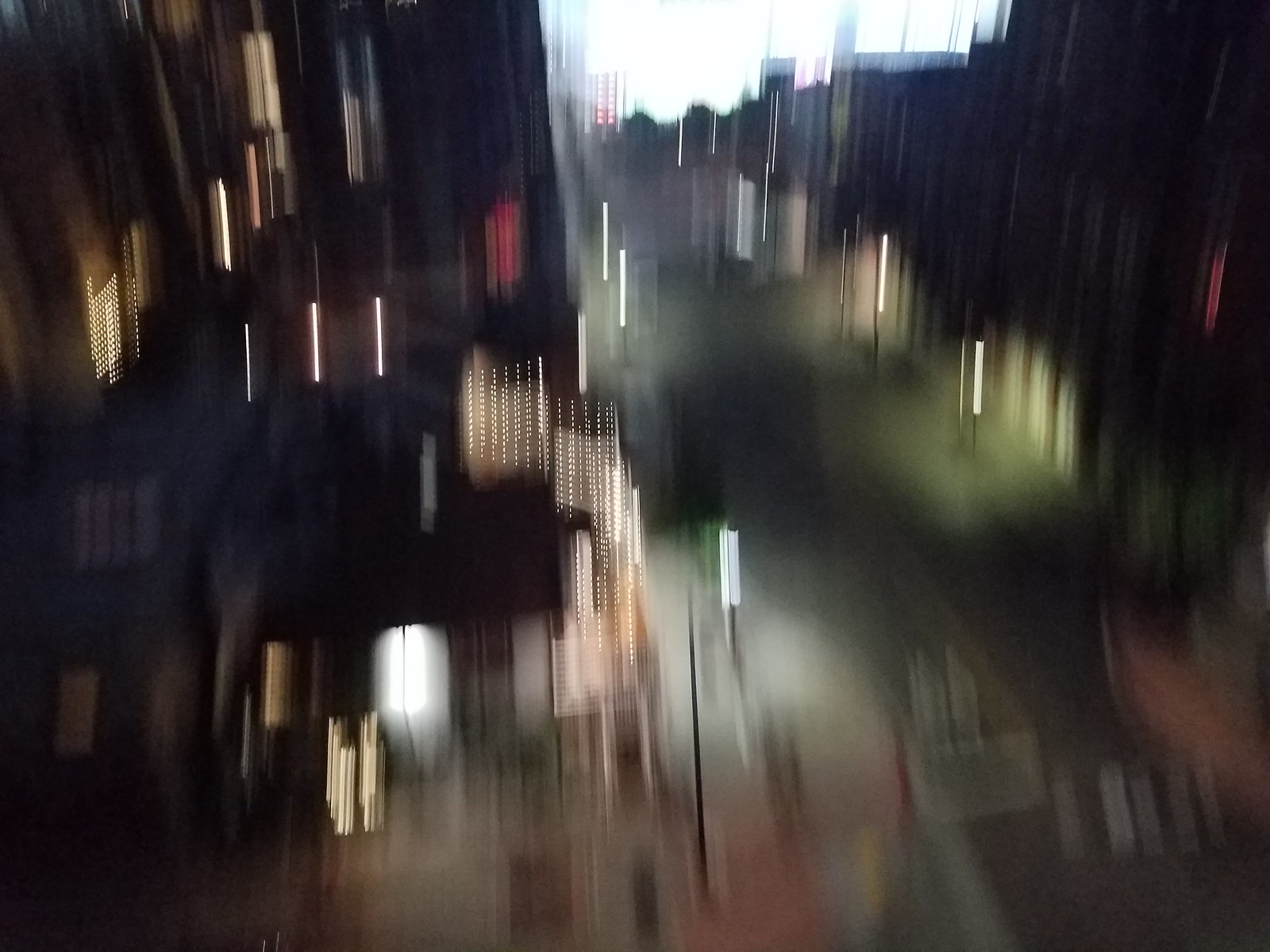The image is a very blurry, out-of-focus picture of a city street, likely taken at dusk or later. The scene is lined by tall buildings on both the left and right sides, possibly apartment buildings about seven or eight stories high. The buildings are predominantly dark with patches of light emanating from streetlights and windows. The streetlights are white and elongated vertically due to the blur, matching the similarly elongated yellow and red lights from the windows and fixtures.

The road runs on the right side of the frame with some illegible white markings. At the top right corner of the image, several buildings reach towards the center, blending into the dominantly white sky background. Streetlights illuminate both sides of the street, and you can distinguish faint, indistinct silhouettes of people moving within the scene, emphasizing the motion blur that makes every detail unclear. Despite the lack of clarity, the image vividly captures the dynamic and illuminated essence of a city street at night.